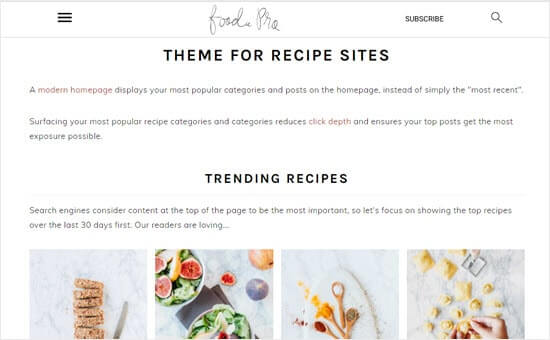This image features a professional-looking food website with a clean layout. At the top of the page, there is a cursive logo—likely saying "Foodie" followed by another indistinguishable word. On the left side of the top banner, there is a hamburger menu icon represented by three horizontal lines. To the right, there is a "Subscribe" button followed by a search icon depicted as a magnifying glass.

Below this white top banner, there is a thin line separating it from the rest of the page content. The banner under the line has bold black text stating, "The theme before recipe sites." Directly below, written in red font, is a tagline that reads, "A modern home page." Further down, there are a couple of lines of additional information indicating a focus on trending recipes. It specifies, "Search engines consider content at the top of the page to be the most important. So let's focus on showing the top recipes over the last 30 days. First, our readers are loving…"

Below this text, four food images are displayed, though they are partially cut off. One image includes a person’s hand at the bottom, while the others solely feature the dishes themselves. The images and the content suggest an emphasis on popular recipes curated for user interest and search engine optimization.